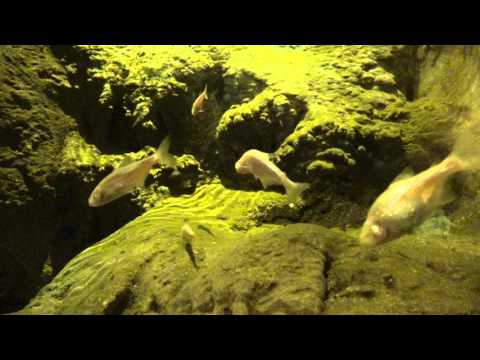The image depicts an underwater scene, possibly in a fish tank, featuring a total of five fish swimming among algae-covered rocks. In the foreground, three goldfish are prominent, appearing larger and more detailed due to their proximity to the camera. Behind them, two smaller fish can be seen, one near the top center and another near the bottom center, adding depth to the scene. The distant fish display a mix of gold and darker orange-gray hues. The background showcases a variety of rock shapes, all enveloped by a thick layer of green moss, contributing to a monochromatic, slightly blurry aesthetic with dark spots that resemble small caves, enhancing the cavernous ambiance. The entire scene is framed by black bands at the top and bottom, giving it a cinematic feel.